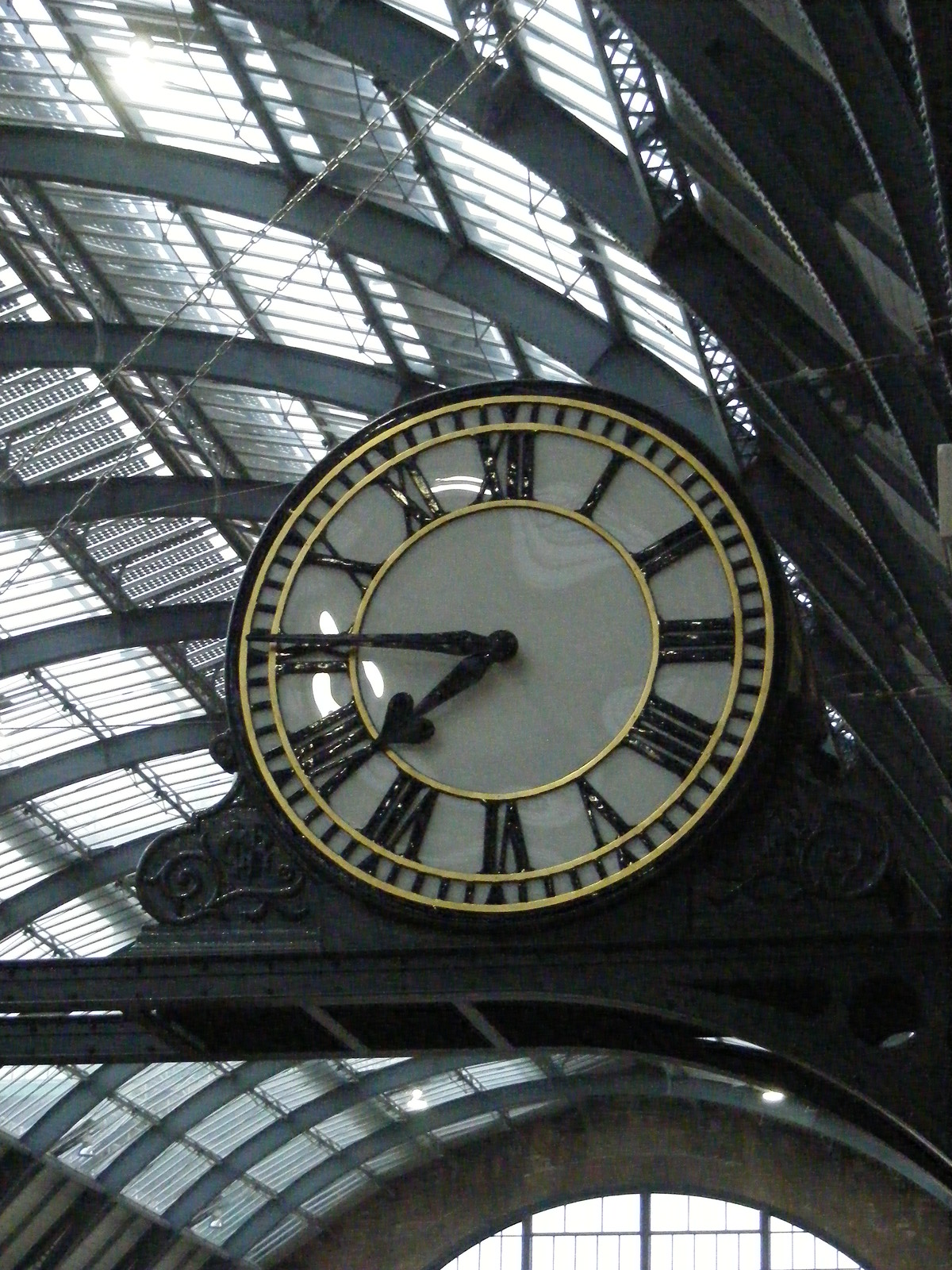This photograph captures the grand interior of a historic building, showcasing an awe-inspiring domed ceiling constructed from elegantly curved, black iron girders. These girders arch gracefully across the ceiling, framing large window panes that allow abundant natural light to flood the space below. In the detailed foreground, there is a visibly intricate clock encased within an elaborate black iron frame adorned with swirling motifs and possibly floral carvings. This ornate clock is mounted on a horizontal iron beam that extends outward, though its terminus is not shown.

The clock's face is pristine white with a glossy finish, featuring prominently visible black Roman numerals marking the hours. The hands of the clock are also black, with the hour hand uniquely designed with a heart-shaped tip and the slender minute hand tapered elegantly toward its end. Surrounding the numerals, minute divisions are indicated by small black lines. Additionally, three small gold circles are painted onto the face of the clock, adding a touch of opulence to its design. This intricate timepiece contrasts beautifully against the expansive, light-filled ironwork and glass ceiling that forms the majestic backdrop of this remarkable interior.